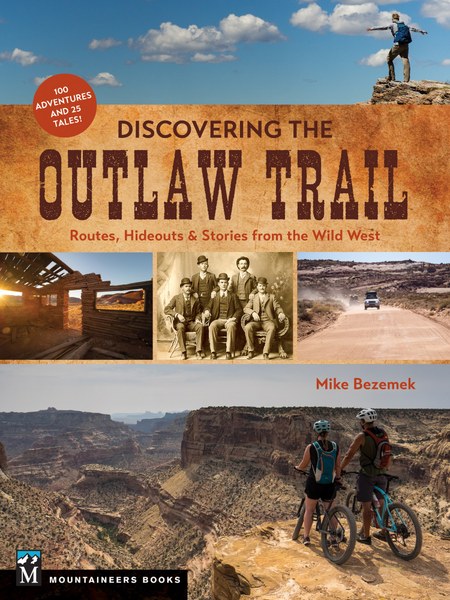The cover of a book titled "Discovering the Outlaw Trail: Routes, Hideouts, and Stories from the Wild West" features a layered design with multiple images and text elements. At the very top, there's a clear blue sky with a few puffy white clouds. On the right side of this sky section, a man stands on the edge of a cliff with his arms outstretched, wearing a blue backpack. Below this scene and taking up a significant portion of the cover is a large aged brown rectangle. In large white letters, it reads "Discovering the Outlaw Trail," while below it in smaller orange text, it says "Routes, Hideouts, and Stories from the Wild West." Slightly above and to the left of the brown rectangle is a white circular bubble stating "100 adventures and 25 tales."

Directly beneath this text section are three photographs: the first on the left shows a blue sky with a wooden cabin under construction, the middle photograph is a sepia-toned image of three men sitting and two men standing behind them, and the third on the right is a more modern-day picture of a truck or SUV on a dirt road with mountains in the background. At the very bottom of the cover is a larger horizontal photograph of two people on mountain bikes at the edge of a steep canyon, possibly the Grand Canyon, looking over the vast landscape. Above this photograph, in orange letters, is the name "Mike Bezemek."

In the lower left-hand corner of the cover, there's a black rectangle featuring a white capital "M" logo with a mountain outline and the words "Mountaineers Books."